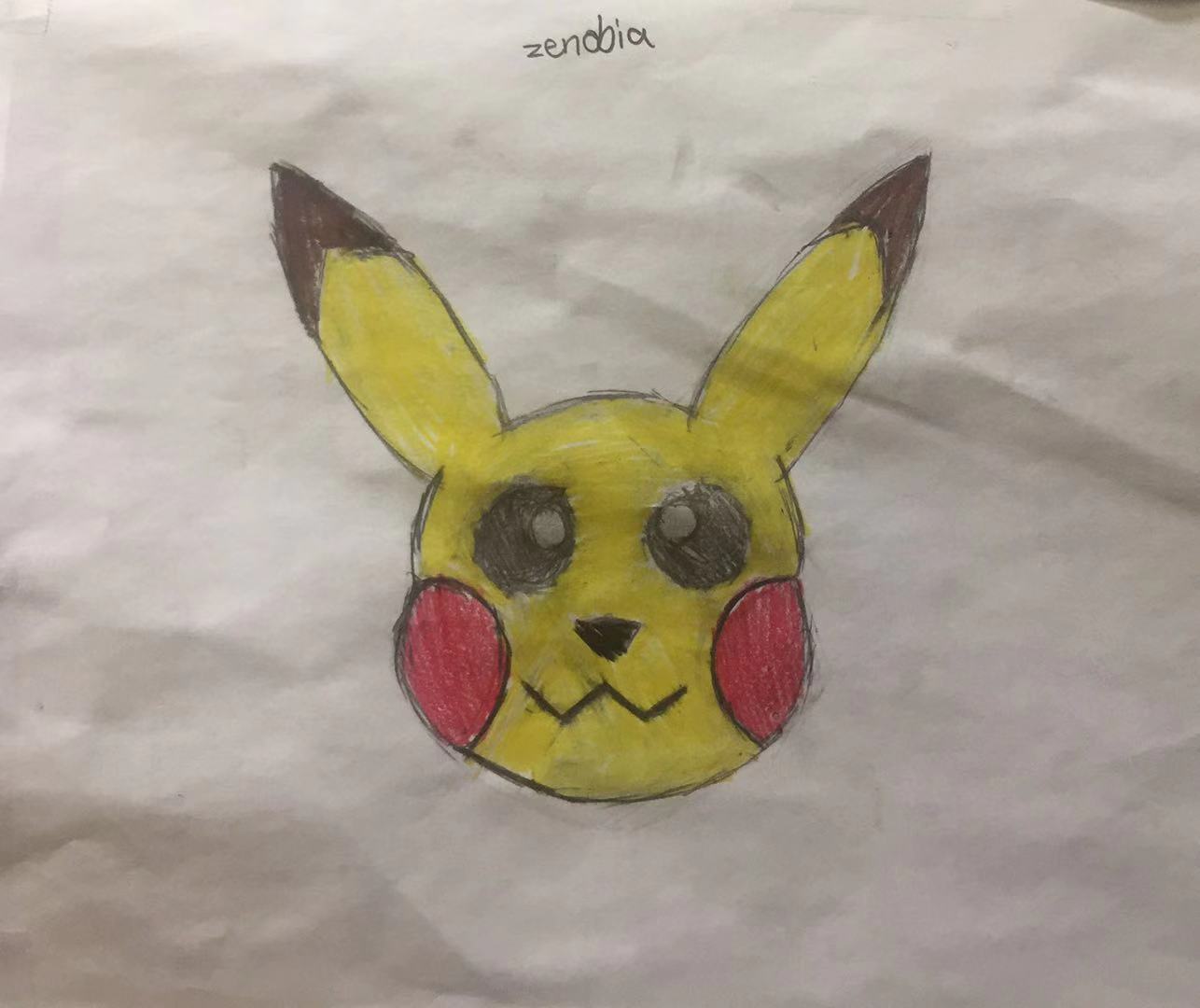The image features a crumpled piece of white paper, which may be from a printer or sketch pad. At the top center of the paper, the name "Zenobia" is printed in black, uppercase letters. The paper itself is heavily wrinkled and creased, with lighter tones at the top and left side, contrasting against its generally grayish appearance.

In the center of the paper is a drawing of Pikachu. Pikachu's head is a bright yellow and round in shape, with two pointy ears that are black at the tips. His large, black eyes are pencil-colored with gray pupils in the center. On either side of his face are two prominent red cheeks, depicted as large circles. Pikachu's nose is a small, upside-down black triangle, and his mouth forms a zigzag, W-shaped pattern.

Overall, the depiction combines hand-drawn elements with the unique texture of the wrinkled paper, adding a distinctive character to the illustration.